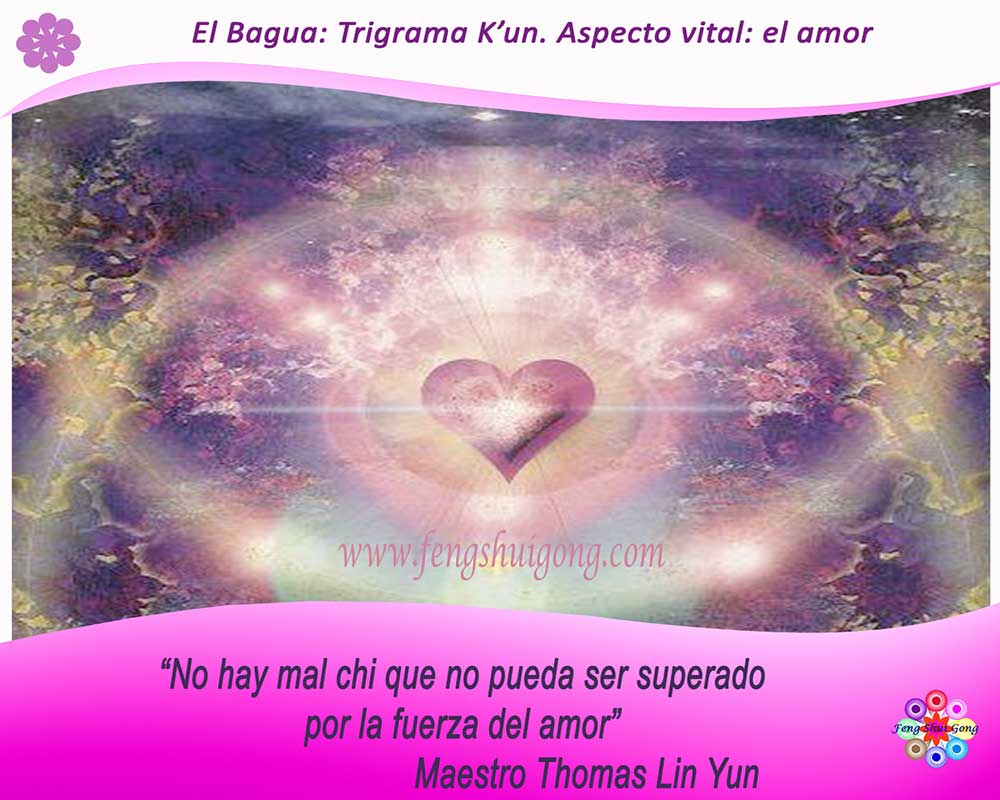The image showcases an artistic heart at its center, radiating rays that form a petal-like pattern. The heart is surrounded by rings of light, set against a detailed, decorative background with shades of blue and aqua. The background also includes hints of a grainy world map or natural landscape of streams and valleys. Below the heart, a swirling mauve or light pink area contains Spanish text that translates to "There is no evil that cannot be overcome by the power of love. Master Thomas Lin Yun." Additionally, the text at the top reads, "El Bagua trigrama con aspecto vital el amor," and the bottom of the image features the URL www.fengshuigang.com. In the lower right-hand corner, there's a logo, adding a finishing touch to this intricately designed image.